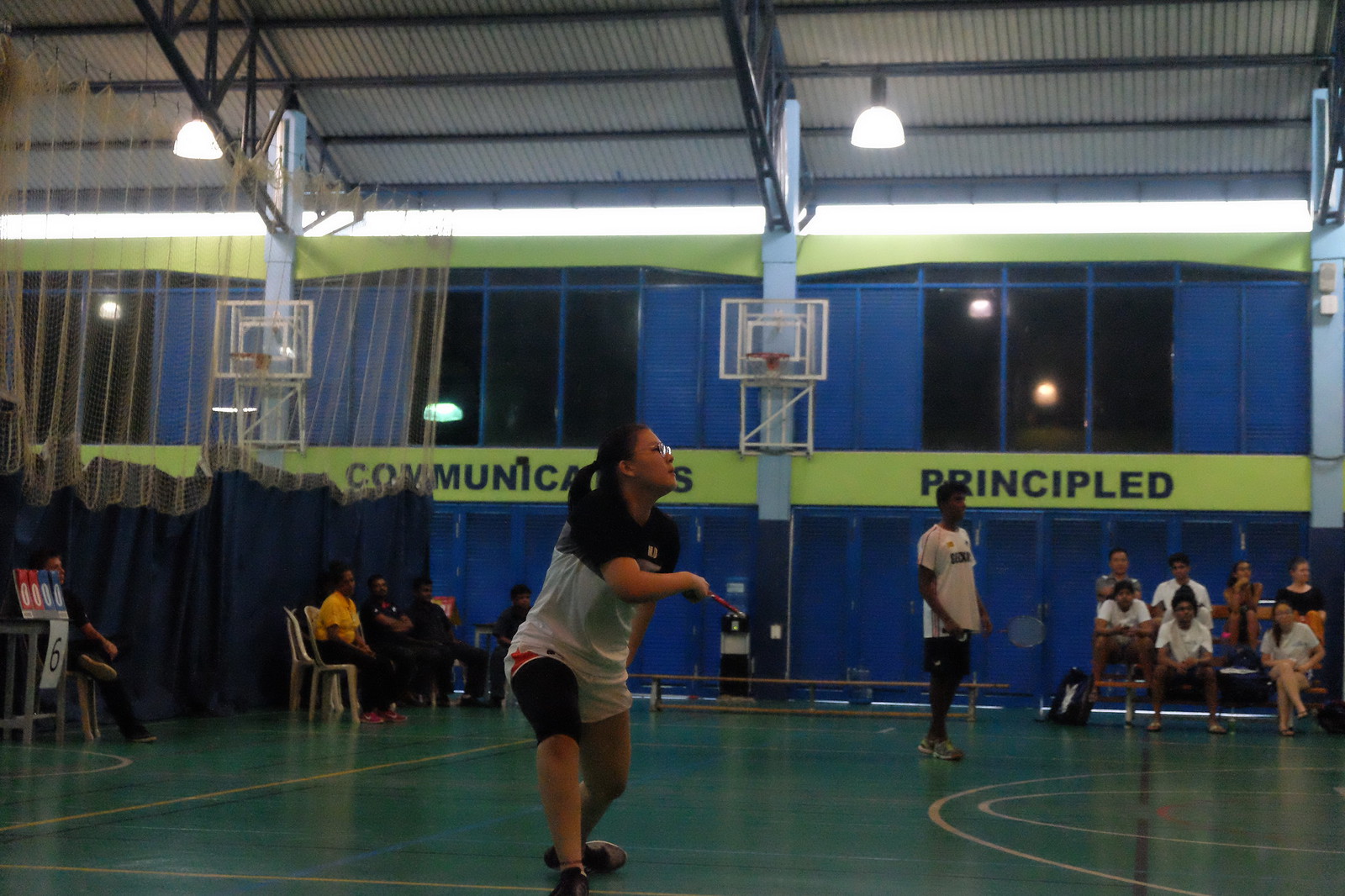The image depicts an indoor basketball court that has been converted into a vibrant badminton court with a green floor and multiple white lines indicating various playing areas. The ceiling is silver with intricate blue support beams and light blue pillars that transition into dark blue padded walls. In the forefront, a woman, dressed in black shorts and a shirt that's black on top and white on the bottom, stands holding a badminton racket. She sports black sneakers with white soles and wears glasses. The focus of her gaze is towards the right side of the image, suggesting she is in the midst of a game. Several people are seated on benches located on both the left and right sides of the court, attentively watching the match. Basketball hoops are visible in the background along with windows at the top of the walls, adding to the gymnasium's multifunctional appeal. The walls bear a yellow banner with the words "communication" and "principled" prominently displayed. The setting, illuminated by bright ceiling lights, indicates a lively indoor environment, most likely during night time.